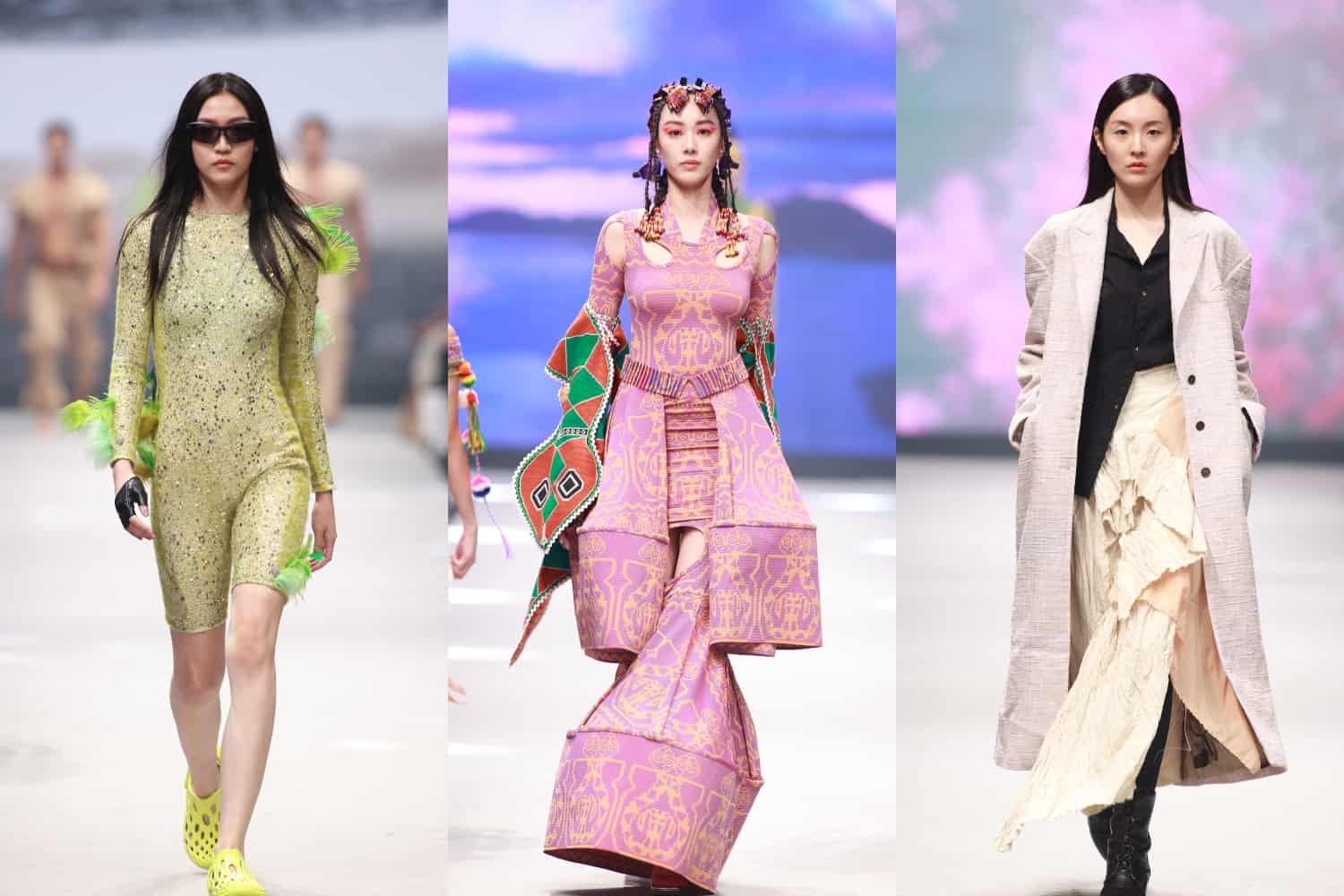In this detailed fashion ensemble, the image is divided into three distinct photographs, all showcasing what appears to be the same woman dressed in three different avant-garde outfits, as if part of a high-fashion runway show.

In the first photograph on the left, the woman dons a form-fitting, green sequin jumpsuit adorned with feathers on the left shoulder, right arm, and left thigh. The jumpsuit, which combines long sleeves with knee-length leggings, also features a speckled pattern of black and white dots. She accessorizes with black fingerless gloves on her right hand and yellow open-weave sandals that resemble Crocs, made from a foam material. Her look is completed with long dark hair and sleek black sunglasses, with two out-of-focus men faintly visible in the background.

The center photograph showcases the woman in a striking pink dress with Oriental influences. The dress hugs her curved waist and has multiple cutout areas around the neck and shoulders. A prominent feature is the tubular, tent-like structure that extends around her lower legs, adding a dramatic flair. She pairs this with a vibrant shawl and heavy white makeup accentuated by pink eyeshadow. Her hair is styled in braids that frame her face, enhancing the overall traditional yet modern aesthetic.

In the photograph on the right, the woman is dressed in a layered, beige flouncy skirt paired with a partially tucked black shirt. Over this, she wears a flowing tan linen overcoat. Her sleek, straight dark hair complements her ensemble, along with her choice of black boots that complete her chic look. This varied yet cohesive series of photographs highlights the versatility and boldness of high-fashion.